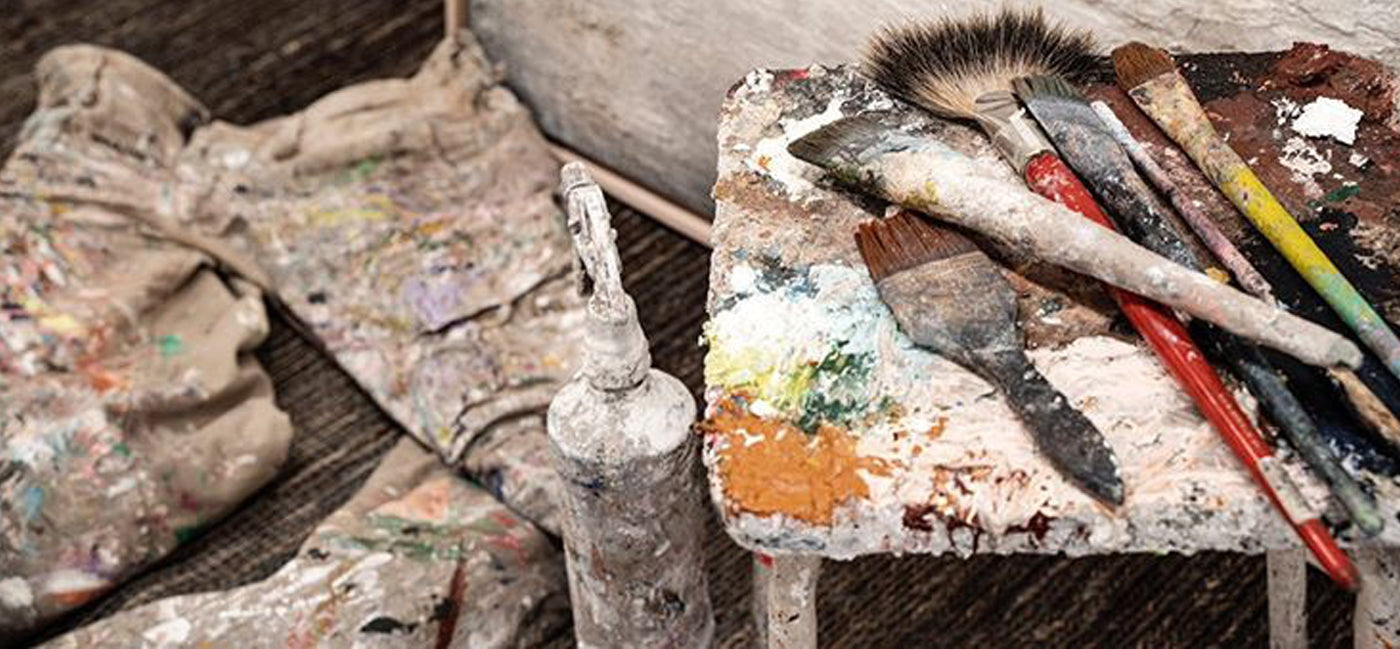In this indoor close-up photograph, a heavily textured and colorful scene unfolds, capturing an artist's workspace saturated with paint. Dominating the right side is a stool thickly coated in layers of paint. Atop this stool rests an array of six paintbrushes of various shapes and sizes, from regular to fan brushes, all similarly encrusted with remnants of old paint in diverse colors. Central to the image is a cylindrical spray bottle, almost camouflaged by its coating of white, gray, and bluish paints, rendering its text and design unrecognizable. To the left, slightly out of focus, lies a crumpled pair of tan pants, similarly splattered with vibrant paint splotches in red, blue, and green. The overall setting is likely an art studio, illuminated in a way that slightly washes out the colors but accentuates the intricate textures and suggests the long-term use of these well-worn tools.